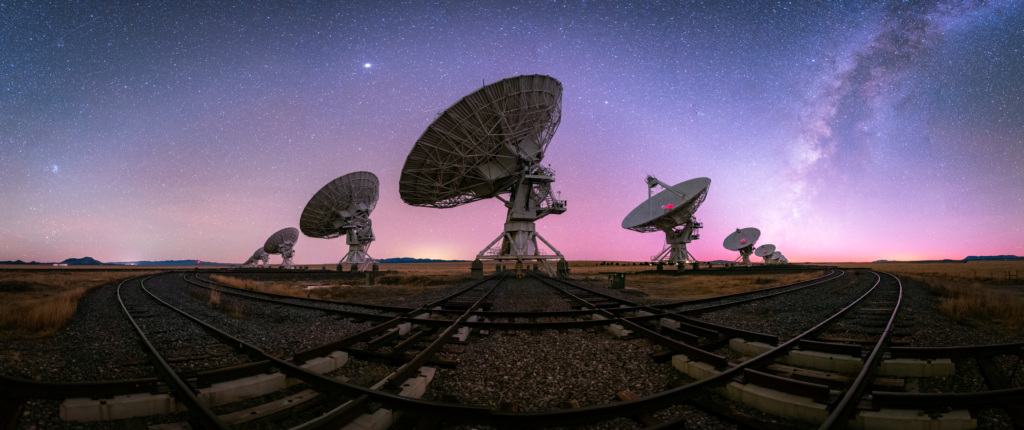This professional, panoramic photograph, taken at night, captures a mesmerizing scene at a crossroads where four sets of railroad tracks meet. Two sets of tracks extend away from the photographer, while the other two run left to right across the image, framed by gray gravel and brown vegetation. The sky is a vibrant gradient, transitioning from darker blue at the top to lighter purple and then to a bright pink near the horizon, indicating that the photograph was taken at sunset in a desert area. The night sky is densely populated with stars, highlighted by the visible arm of the Milky Way galaxy in the upper right corner. The main focal point is an array of very large, metal radio satellite receivers, arranged in a U-shape, each pointing at different angles toward the star-studded sky. The long exposure used in capturing this image intensifies the star density, creating a striking contrast with the impressive silhouette of the satellite dishes.